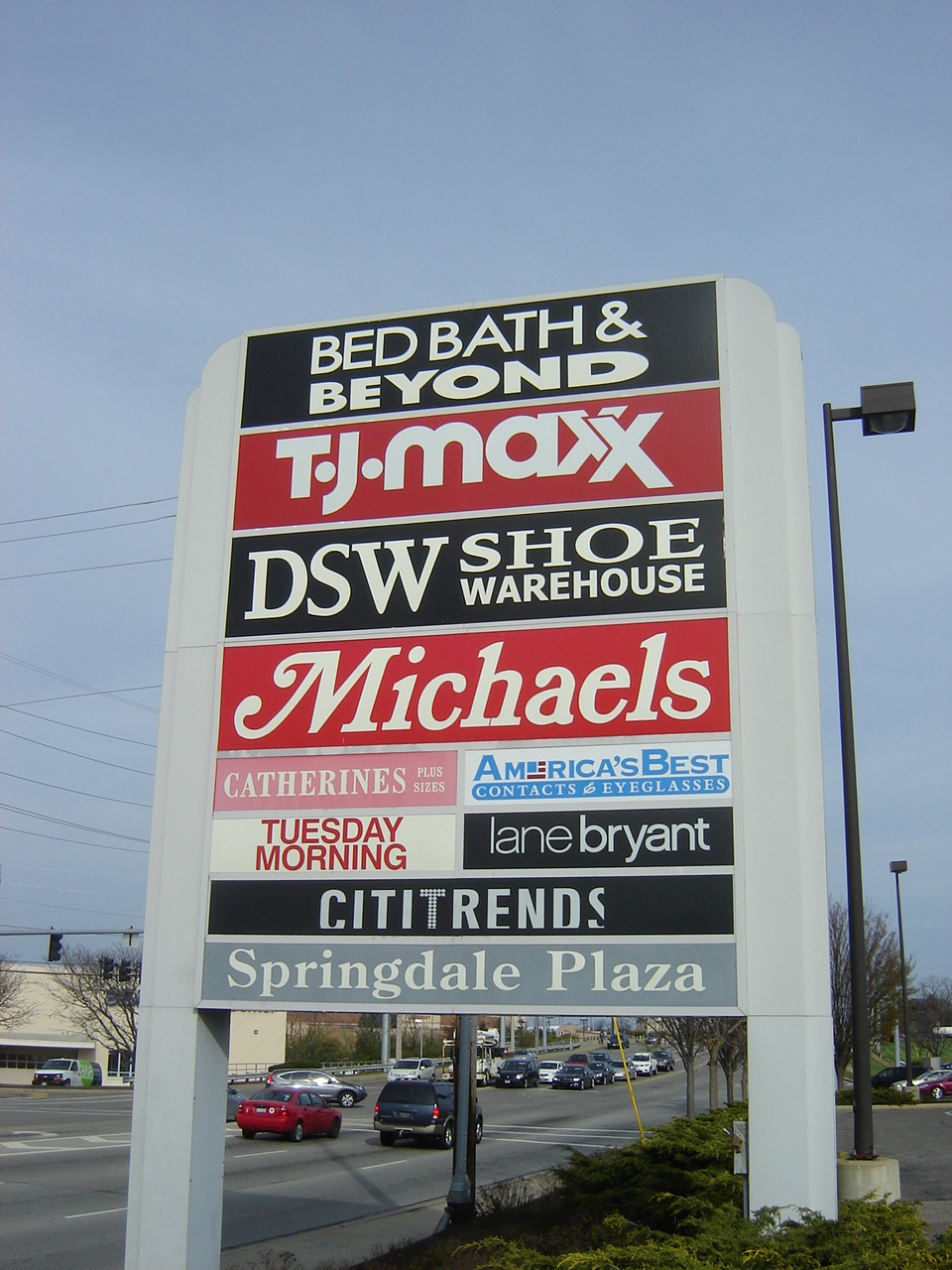This is a detailed photo of a large sign outside Springdale Plaza, a bustling shopping center along a busy, multi-lane street with visible traffic and a grassy lot surrounding the base. At the top of the sign, a black banner with white letters announces "Bed Bath & Beyond." Below it, a red banner with white letters says "TJ Maxx," followed by "DSW Shoe Warehouse" on another black banner with white letters. Next is "Michaels" on a red background with white lettering. The next line features two smaller signs: "Catherine's Plus Sizes" on the left with white lettering on a pinkish-red background, and "America's Best Contacts and Eyeglasses" on the right, in blue letters on a white background. Below these, "Tuesday Morning" is written in red letters on a white banner on the left, and "Lane Bryant" in white letters on a black background on the right. The line below lists "City Trends" in white letters on a black background. Finally, at the bottom, "Springdale Plaza" is prominently displayed in large white letters on a bluish-gray background. Two tall streetlamps are visible beside the sign, with one positioned closer to the picture. The vibrant, blue sky and the busy roadway with multiple cars and possibly a bus underscore the lively atmosphere of this retail hub.